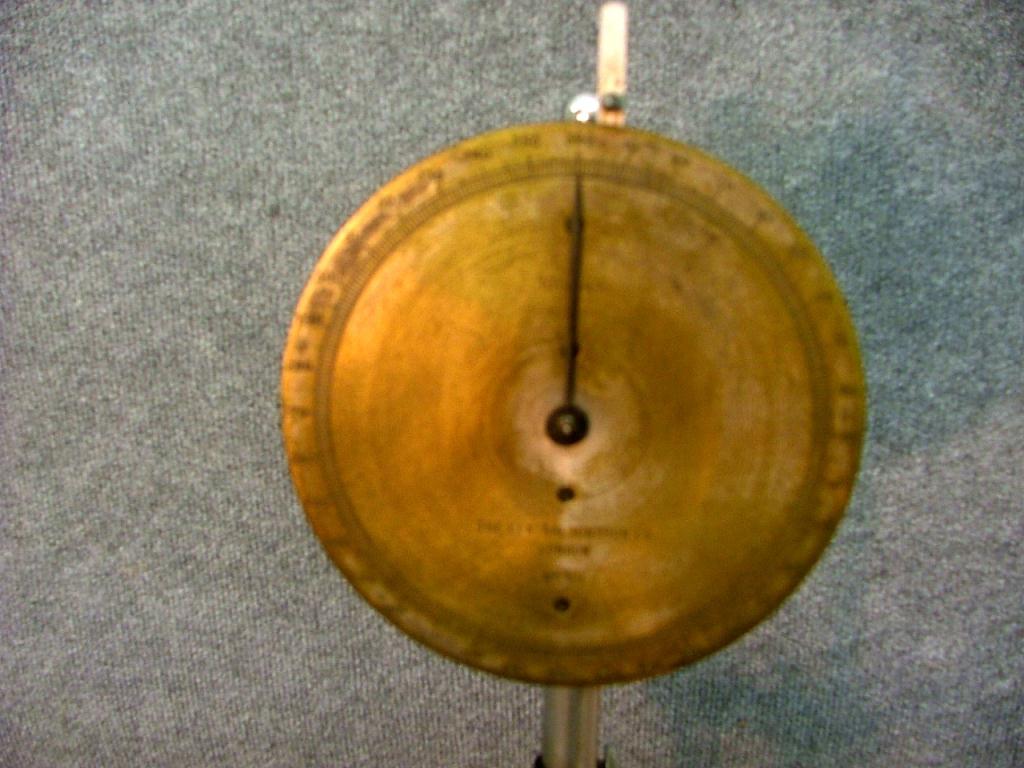The close-up image showcases a vintage, rusted dial that exhibits a mix of faded yellow and brown hues. The dial is circular with a slightly visible section of a gray pole at the bottom, indicating its support structure. The face of the dial features fragmented black text near the center, flanked by circular black markings at the top and bottom. At the heart of the dial, there is a prominent black circular element, from which a needle extends vertically upward. Just to the right of this needle, a small, vertical stick-like feature with a black dot in its center can be observed, illuminated by a soft light. The backdrop of the image is primarily a light gray, rug-like texture, punctuated by patches of blue on the right and lower edges.